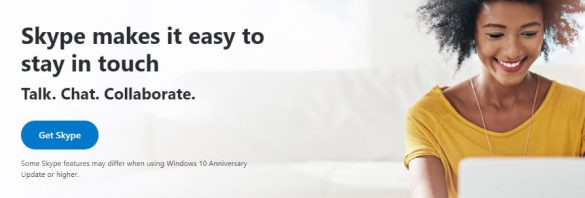The image showcases a modern advertisement for Skype, set against a light gray background. Prominently in the background is a bright, white, illuminated window. The central message in black text reads, "Skype makes it easier to stay in touch, talk, chat, collaborate." Below the text, a vibrant blue button with white text prompts viewers to "Get Skype."

In the lower part of the image, there is a smiling Black woman with voluminous hair. She’s adorned with a gold chain and is wearing a bright yellow shirt. The woman is engaged and appears to be looking down at a white computer, perhaps using Skype. The image introduces additional context noting, "Some Skype features may require Windows 10 Anniversary Update or higher."

Overall, the advertisement effectively positions Skype as a user-friendly tool for communication and collaboration, illustrated by the joyful user immersed in her interaction on the platform.